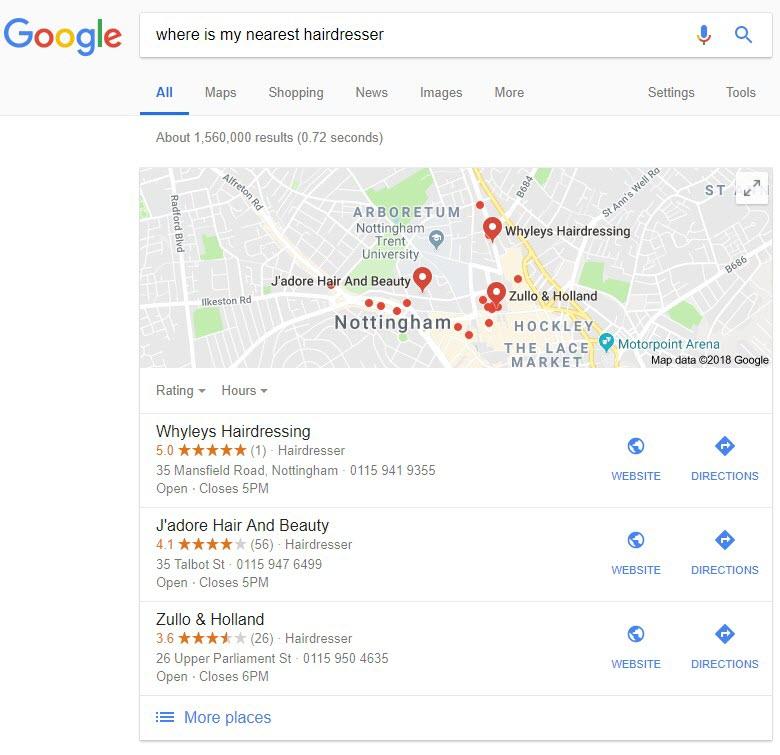This image is a screenshot of Google search results for the query "where is my nearest hairdresser." At the top, Google's iconic logo is prominently displayed. The search bar contains the typed query, and directly below it, there is a menu bar offering various search options: All, Maps, Shopping, News, Images, More, along with Settings and Tools. The "All" option is highlighted, indicating a search across all categories.

Just beneath this, the search results indicate there are approximately 1,560,000 results generated in 0.72 seconds. Below this summary, a map of the surrounding area is displayed, marked with several red dots that pinpoint the locations of nearby hairdressers. Some of these locations are further highlighted with bubble icons displaying their names, potentially signifying paid promotions for increased visibility.

Further down, there are detailed listings for three hairdressers: Wiley's Hairdressing, J'Adore Hair and Beauty, and Zulo in Holland. Each listing includes a rating, category (hairdresser), address, phone number, current open status with closing times, website link, and directions. At the bottom of the screenshot, there is an option to click for a "More places" menu, likely to see additional results beyond the initial three highlighted on the map.